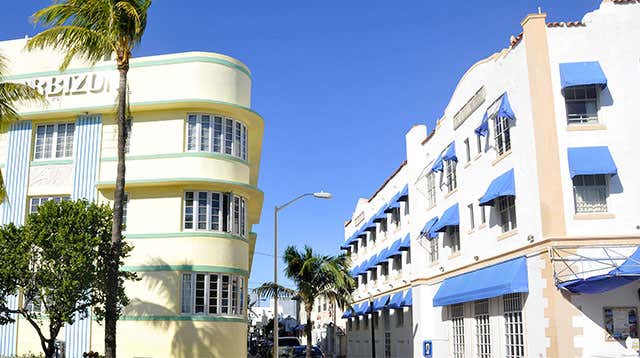Captured from an elevated vantage point, this image presents a vibrant street scene flanked by two distinctive buildings in a tropical locale, underscored by the presence of palm trees. On the left, we see a corner building of ovular shape, adorned with the partially visible sign "ARBIZO." The structure is characterized by its tannish-brown facade, accentuated with vertical blue lines and green horizontal bands demarcating different levels. A tall palm tree with lush green leaves stretches upwards, nearly extending beyond the photo's top border, accompanied by a shorter tree with dense foliage at its base.

Dominating the right side of the image is a white building distinguished by its blue awnings shading each window, suggestive of a hotel or apartment complex. This building extends deeply back and features brown pillar columns that provide subtle architectural contrast. Between the two structures, a street lamp stands out in the middle ground, adding depth to the scene. Smaller elements such as parked and possibly moving cars are faintly visible, enhancing the dynamic cityscape. The sky overhead is clear and blue, completing the picturesque snapshot of this bustling, tropical street.